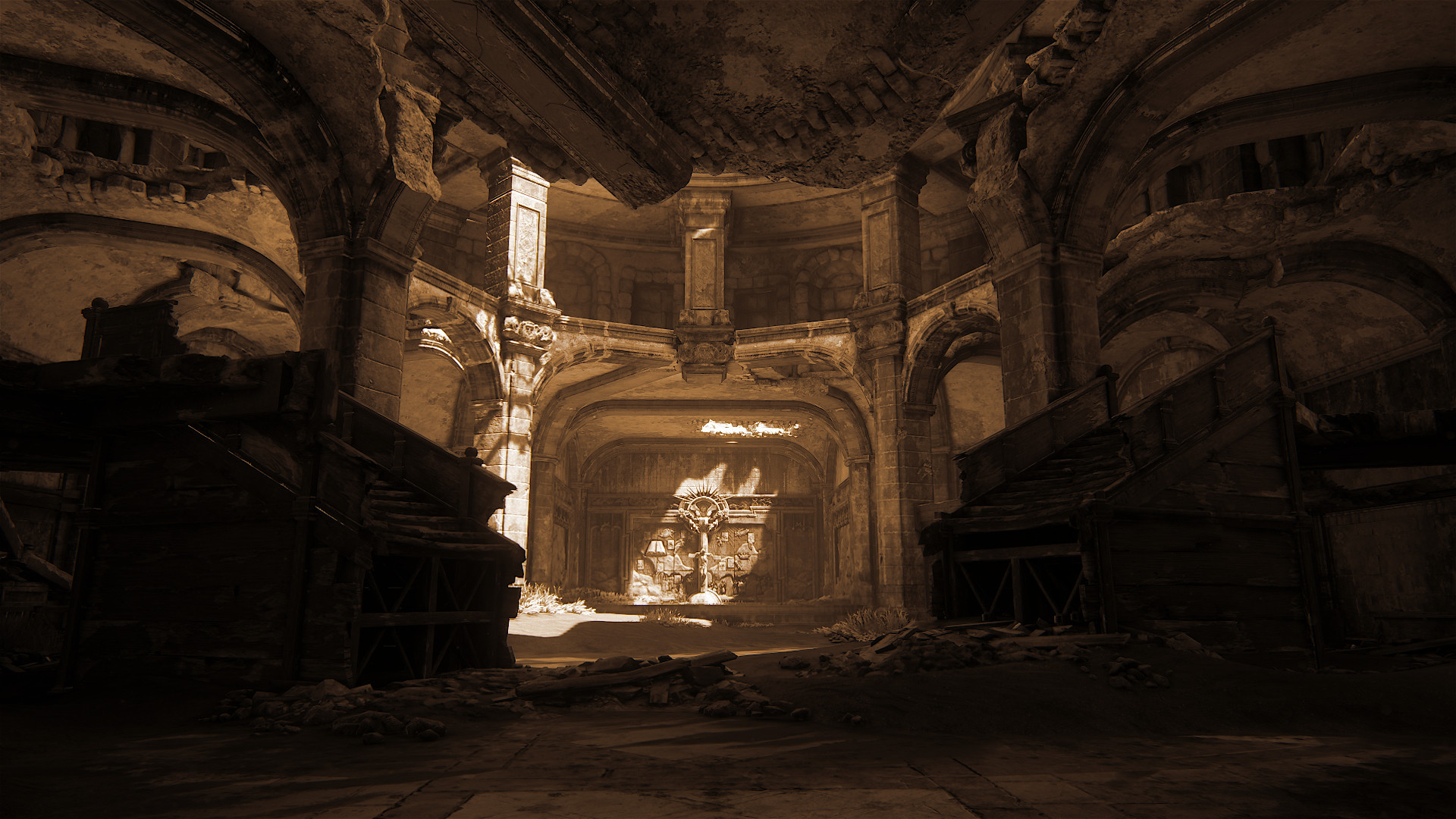The image appears to be a highly detailed shot from a video game, depicting the ruins of an ancient, almost Colosseum-like structure, possibly Greek. The interior suggests a vast, crumbling building with tall, two-story concrete walls etched with unreadable carvings that fade into the back. Sunlight streams in from the top left, illuminating the decaying remnants within. The foreground remains shadowed, littered with debris, broken stairwells, and rubble on the ground. Among the crumbling columns and deteriorating ceiling stands a massive wooden door adorned with ironwork, adding an air of imposing grandeur to the ancient ruins.